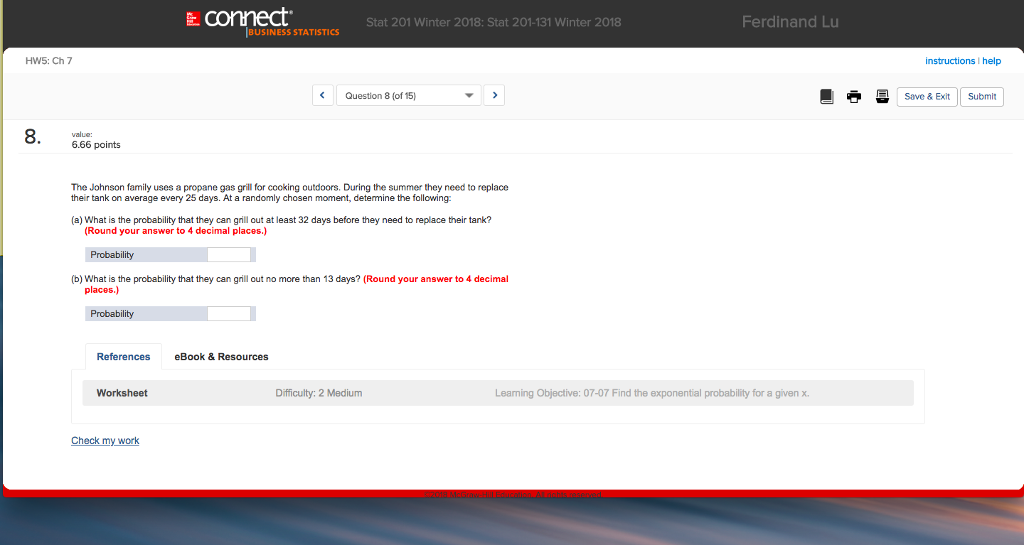**Detailed Caption:**

This image depicts a screenshot from a widescreen desktop or laptop display, specifically showing a page from "Connect Business Statistics." The top of the interface features a dark gray header with "Connect" prominently displayed in white text. Beneath this header, "Business Statistics" is written in bright orange text. In the upper-right corner, the name "Ferdinand Liu" is displayed.

The majority of the background is light-colored, providing a contrast to the navigation elements. There are navigation arrows on the left and right sides of a drop-down menu box, indicating that the page is currently on Question 8 out of a total of 15. Users have the option to navigate to previous or subsequent questions using these arrows.

Below the navigation section, there is information about the current question: "Question 8 of 15," specifying that this question is worth 6.6 points. The detailed question text reads:

"The Johnson family’s appropriate gas grill is for cooking outdoors. During the summer, they need to replace their tank on average every 25 days. At a randomly chosen moment, determine the following:

A) What is the probability that they can grill out at least 32 days before they need to replace their tank? (Round your answer to four decimal places.)

B) What is the probability that they can grill out no more than 13 days? (Round your answer to four decimal places.)"

The requirements for rounding answers to four decimal places are emphasized in red text.